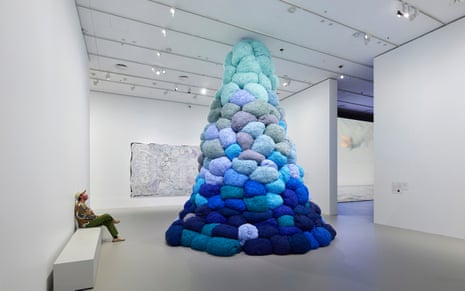In the center of this modern, white-walled art gallery, a striking, large installation commands attention. The room, characterized by its towering height and sleek, contemporary design, is bathed in light from adjustable tracks on the white ceiling. Along the left wall, a white bench supports a man dressed in olive pants, a colorful, printed shirt, and a khaki baseball hat, who sits with crossed legs, gazing up in awe. His gaze follows a towering structure of pillows that narrows as it ascends, transitioning from deep dark blues and purples at the base to progressively lighter shades of blue and purple at the top. The far wall features an indistinct painting, barely discernible in its minimalistic hues of white and light purple, enhancing the ethereal atmosphere. This juxtaposition of the soft, visually captivating mountain of pillows and the man's contemplative pose captures a moment of serene admiration within this expansive, light-filled space.